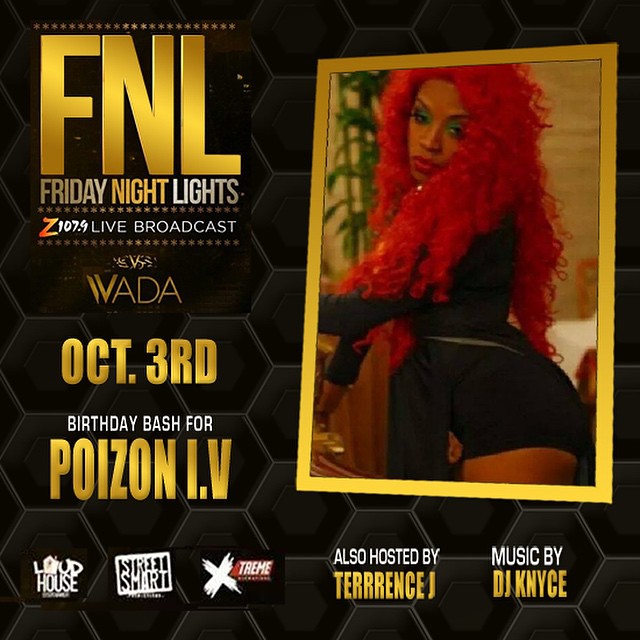The graphic design poster highlights a vibrant birthday bash with a sophisticated layout. Dominating the left side are the large gold letters "FNL," followed by "Friday Night Lights" in smaller font where "Friday" and "Lights" are in white and "Night" is in gold. Beneath that, it reads "Z107.9 Live Broadcast" in white, and further below, "VADA" in gold, with "Oct 3rd, October 3rd" also in gold. Beneath this are the words "Birthday Bash 4" in white and "Poison IV" in gold. 

On the right side of the poster, a striking photo of a woman, likely an African American, with long, bright red curly hair is prominently featured. She's wearing a black dress and has green mascara on. The image captures her from a side profile looking down, with a green plant and a brown wall in the background. This entire section is framed in gold. 

At the bottom of the poster, several logos are displayed, including "Loud House" in white, "Street Smart" in a white square with white text, and "Xtreme" with a spray-painted "X" followed by "treme." The bottom right section indicates that the event is also hosted by Terrence J and features music by DJ Nice, with both names in gold and the accompanying text in white.

The background of the design is a honeycomb pattern in black with white borders, giving it a sleek, modern look.